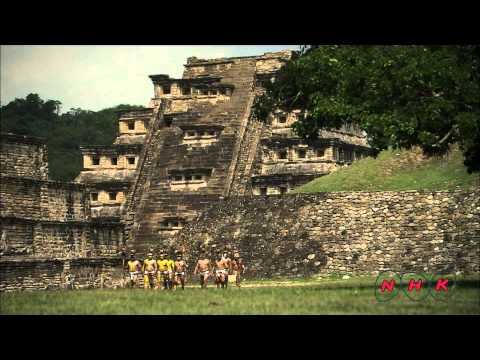This image, which has a vintage feel as if captured on a film camera, depicts a large, ancient stone structure situated on a grassy ground. The main building, resembling a grand library or an ancient temple, is composed of multiple layers and levels with numerous glassless square windows. The central part of the building appears blackened with age, contrasting with the beige sections that remain. A large, slanted piece of gray stone connects to a tall stone wall in front of the building. The complex looks reminiscent of Machu Picchu or Mayan architecture, though it does not resemble a fort. In front of this structure, there is a group of more than five shirtless men walking forward across the green grass. Some of these men appear to be painted yellow and might be wearing tribal attire. In the background, trees are visible, and to the right, a grassy hill peeks over the wall. The letters "N, H, K" appear in red writing in the bottom right corner of the image.